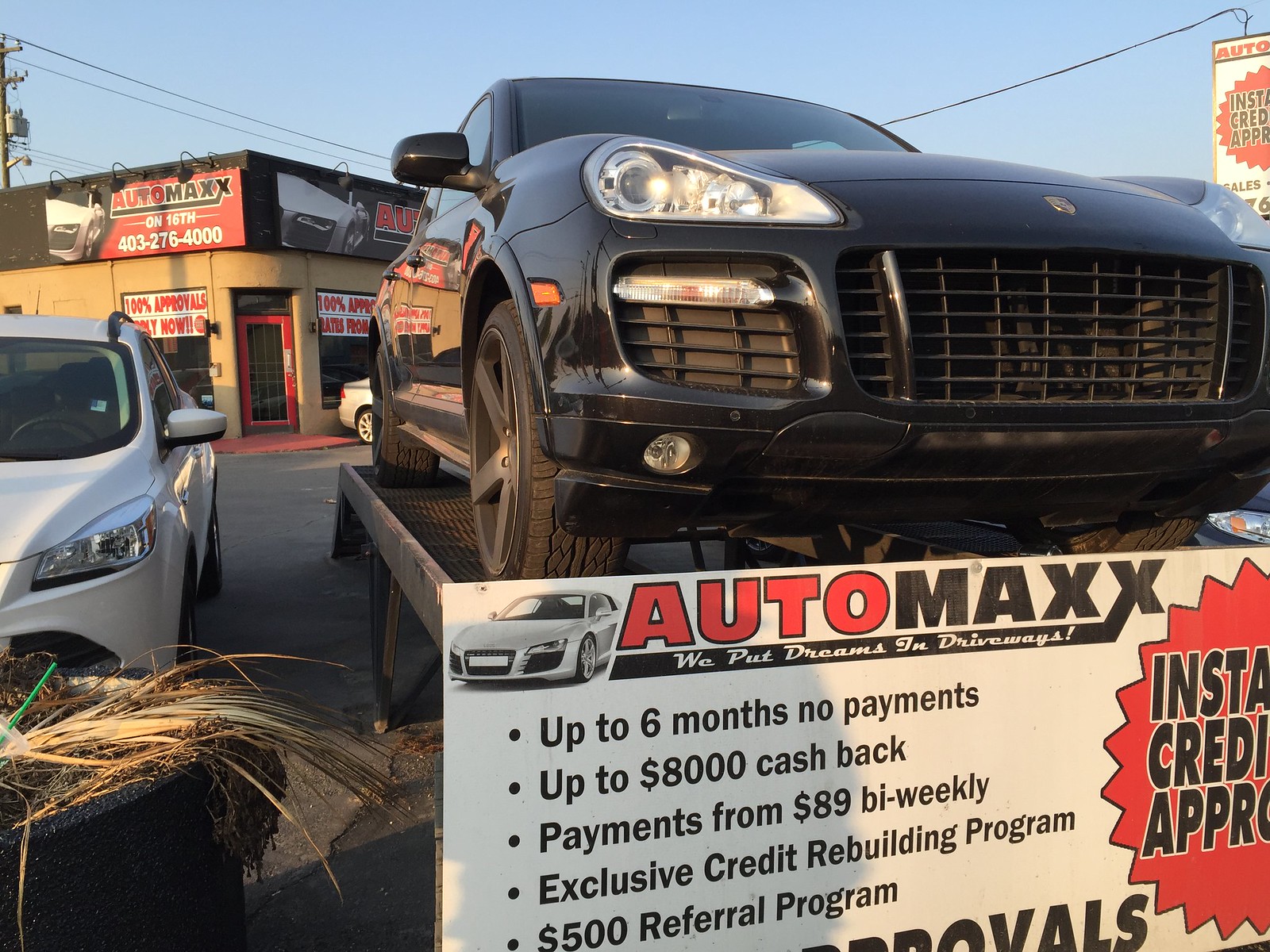The image depicts a parking lot of an American used car dealership named AutoMax. Dominating the scene, a black Porsche Cayenne is elevated on a tow dolly at the front of the lot. In front of this vehicle, a large sign prominently displays various enticing offers: "AutoMax - We put dreams in driveways," "Up to six months no payments," "Up to $8,000 cash back," "Payments from $89 bi-weekly," "Exclusive credit rebuilding program," and "$500 referral program." Additionally, a red badge on the right side of the sign highlights "Instant credit approval."

To the lower left of the display is the front end of a white sedan, while in the background, a dealership building with a red door is visible. This building also bears the AutoMax name and features signage on its windows stating "100% approvals" and "Apply now." Overhead, power lines stretch across a clear blue sky, indicating the photograph was taken outdoors during the daytime. A section of another sign on the upper right corner reads "Auto" and "Instant credit approval," reinforcing the dealership’s promotional messages.